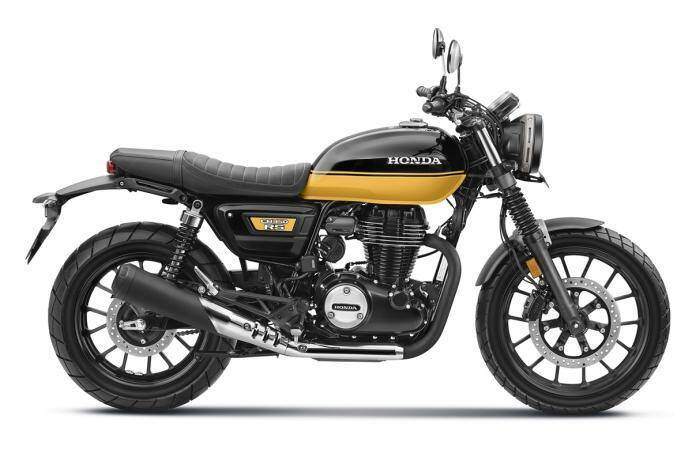The image displays a vintage Honda motorcycle, possibly from the 1970s, set against a pristine white background with its shadow underneath. The gas tank, which is small and rounded, features a distinctive two-tone design: the upper half is black with the Honda name emblazoned in white block letters, while the bottom half is a mustard yellow with thin, reversed black and gold stripes that accentuate the colors. This intricate striping provides a detailed contrast.

The motorcycle seat appears to be a small leather unit with a pattern reminiscent of alligator skin, seemingly designed for two passengers. Just below the seat, there's a side plate with a gold background and white lettering, though the exact text is unclear; it might read "350" and possibly "R5" or "CH-350 R5." Attached to the bottom of the seat is a mud deflector that extends over part of the rear tire.

The bike's exhaust system starts with a black section, transitions to a chrome middle, and flares out into a matte black end. The front end features the classic headlamp and instrument panel, with no additional fairing, accompanied by two round rearview mirrors mounted on rods extending from the handlebars. Notably, the tires have mismatched patterns: the front tire displays a crisscross pattern, while the back tire has a thicker geometric design.